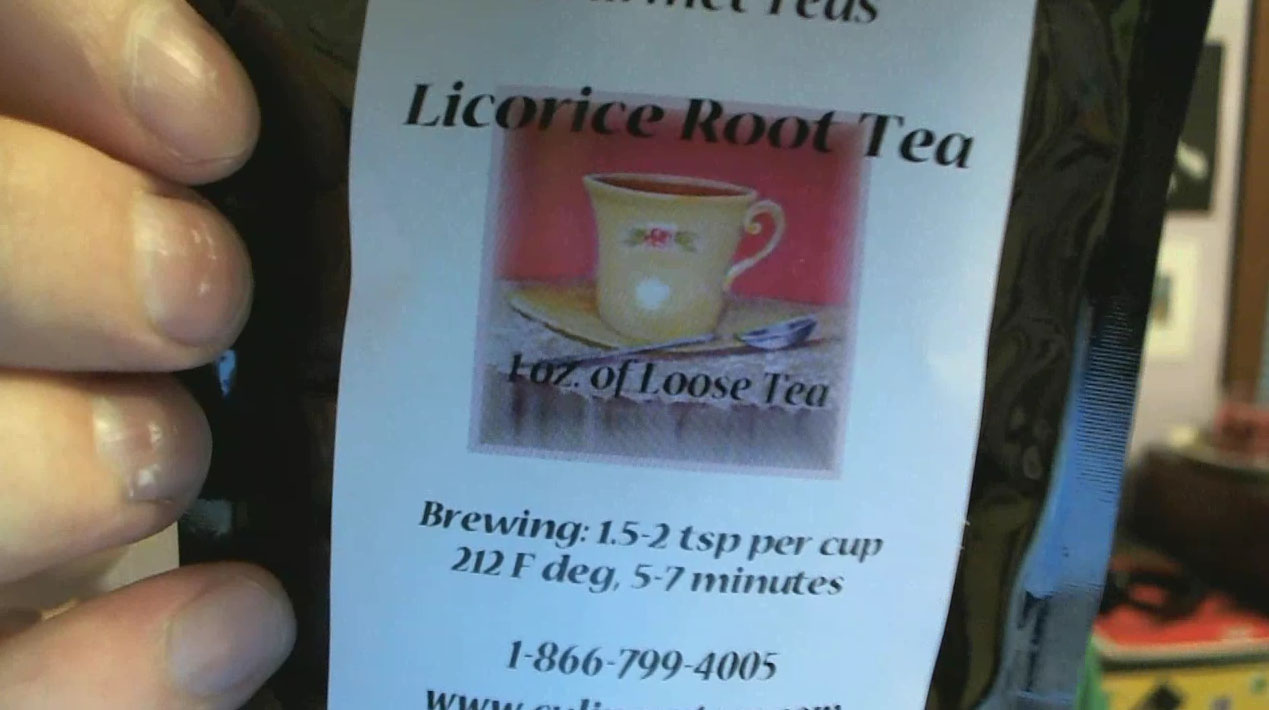In this detailed photograph, a person is holding a dark-sealed plastic packet containing licorice root tea leaves. The person's right hand is visible, with four fingers grasping the right-hand side of the packet. The packaging showcases a white label with black text prominently displaying "Licorice Root Tea." At the top of the label, some text is partially cut off, only revealing the word "teas." 

The label features an image of a yellow tea cup placed on a table with a teaspoon in front of it, all set against a vibrant red background. Below this image, the label provides a description in black text on a white field, stating "One ounce of loose tea." Further brewing instructions specify using 1.5 to 2 teaspoons per cup, with a recommended brewing temperature of 212°F and a steeping time of 5 to 7 minutes. Additionally, a phone number, 1-866-799-4005, is printed below the instructions. A web URL is also mentioned but is partly obscured at the bottom of the photo, making it unreadable.